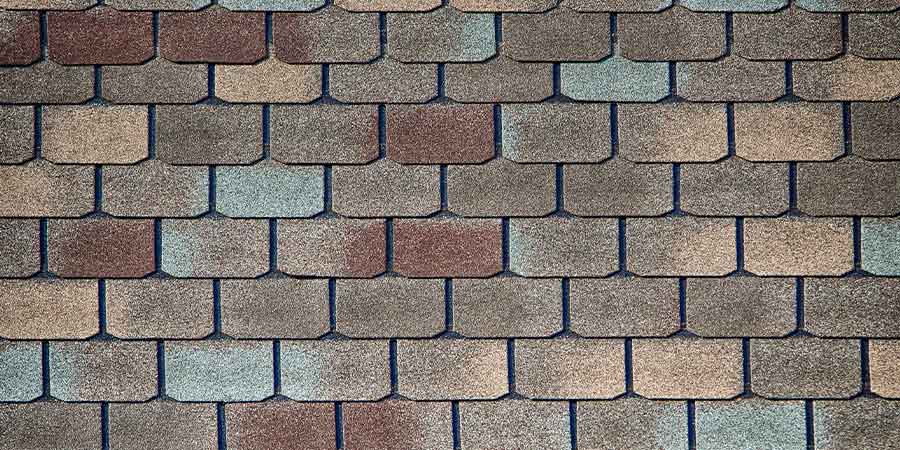This image showcases a meticulously arranged stone pattern, which appears to be part of either a wall or the ground. The repeating pattern consists of nine distinct rows of stones. Each stone exhibits a combination of flat tops and rounded corners at the bottom, giving the layout a visually striking appearance. The stones come in a variety of colors, including shades of brown, gray, yellow, and blue, each featuring a characteristic stone texture. The stones are separated by thin lines of dark black grout, which accentuates their unique shapes and colors while adding to the overall symmetry and neatness of the pattern.